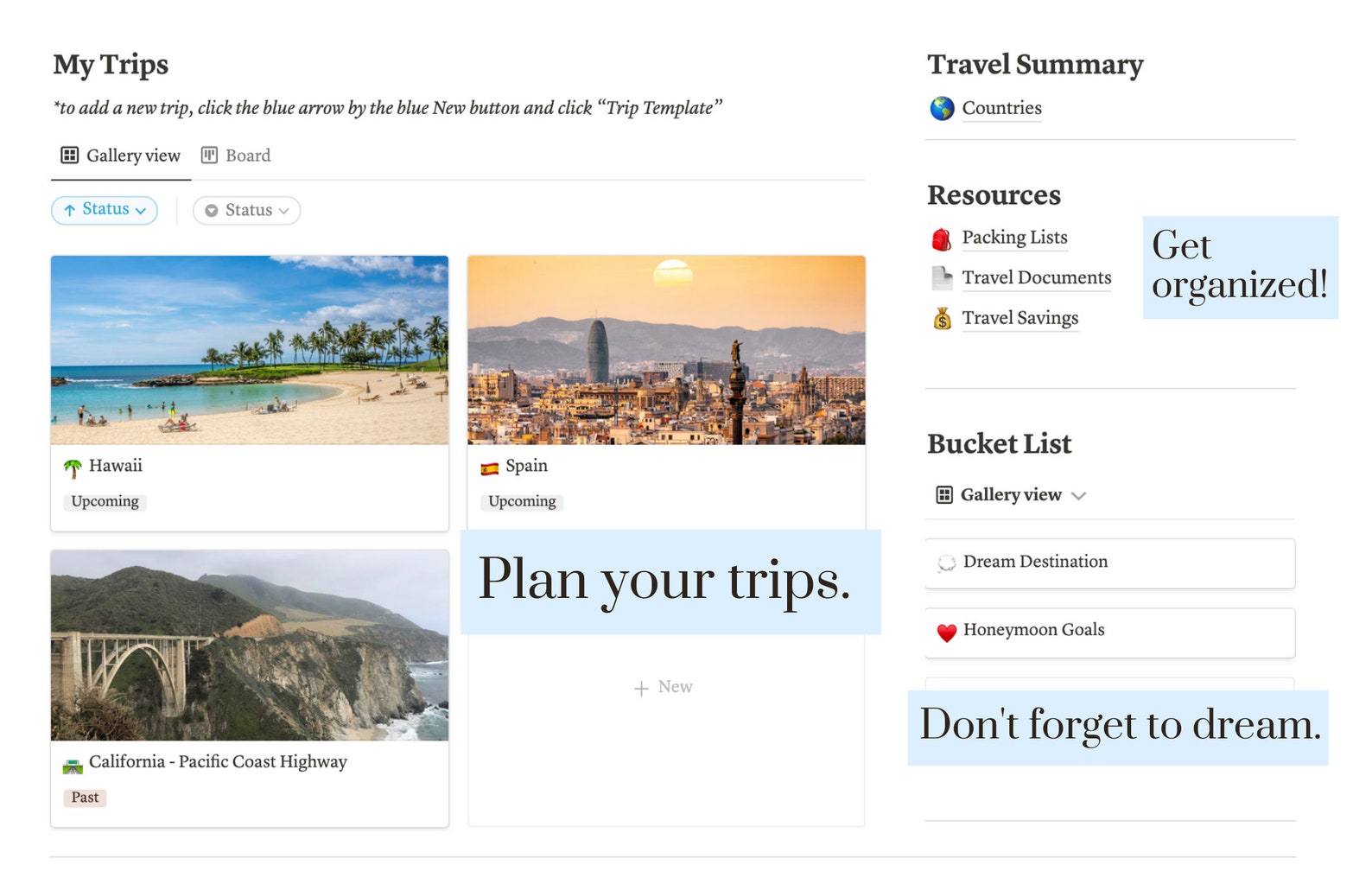This screenshot of a web page features a comprehensive interface from "MyTrips". At the top-left corner, "MyTrips" is displayed in bold black text, while the right side features "Travel Summary" also in bold black. Under "Travel Summary", there is a "Countries" section represented by a globe icon. Proceeding to the "Resources" category, it highlights several items: "Packing Lists" with a red backpack icon, "Travel Documents" with an icon resembling a curled page, and "Travel Savings" accompanied by a money bag with a dollar symbol.

To the immediate right of these categories, there’s a light blue box labeled "Get Organized". Below that, the "Bucket List" section is introduced, starting with "Gallery View" indicated by a grid icon and accompanied by a dropdown arrow. The next item, "Dream Destination", has a faint, indeterminate icon to the left, followed by "Honeymoon Goals" marked with a red heart icon.

Prominently displayed in large black font against a light blue background, the motivational phrase "Don't Forget to Dream" encapsulates the page's inspirational tone. On the left two-thirds of the screen, an instructional note states: "To add a new trip, click the blue arrow by the blue 'New' button, and click 'Trip Template'."

Beneath this, two viewing options are presented—"Gallery View", which is highlighted, and "Board". In the "Gallery View" section, there are two "Status" filters, with the first one being active. Three trip previews are displayed here: 

1. **Hawaii** - This image shows a small cay with a beach, lush greenery, and palm trees. About 20 people are dispersed across the beach and water. This trip is marked as "Upcoming".

2. **Spain** - Featuring numerous stucco houses visible from an aerial perspective with two tall structures—the foreground structure being a pole. The backdrop has mountainous terrain under an orange sky with a visible sun, also marked "Upcoming".

3. **California Pacific Coast Highway** - Depicting a Rocky Mountain area with an ocean-view bridge, this trip is labeled "Past". 

Finally, at the bottom of the screen, the call to action "Plan Your Trips" encourages users to engage with the platform further.